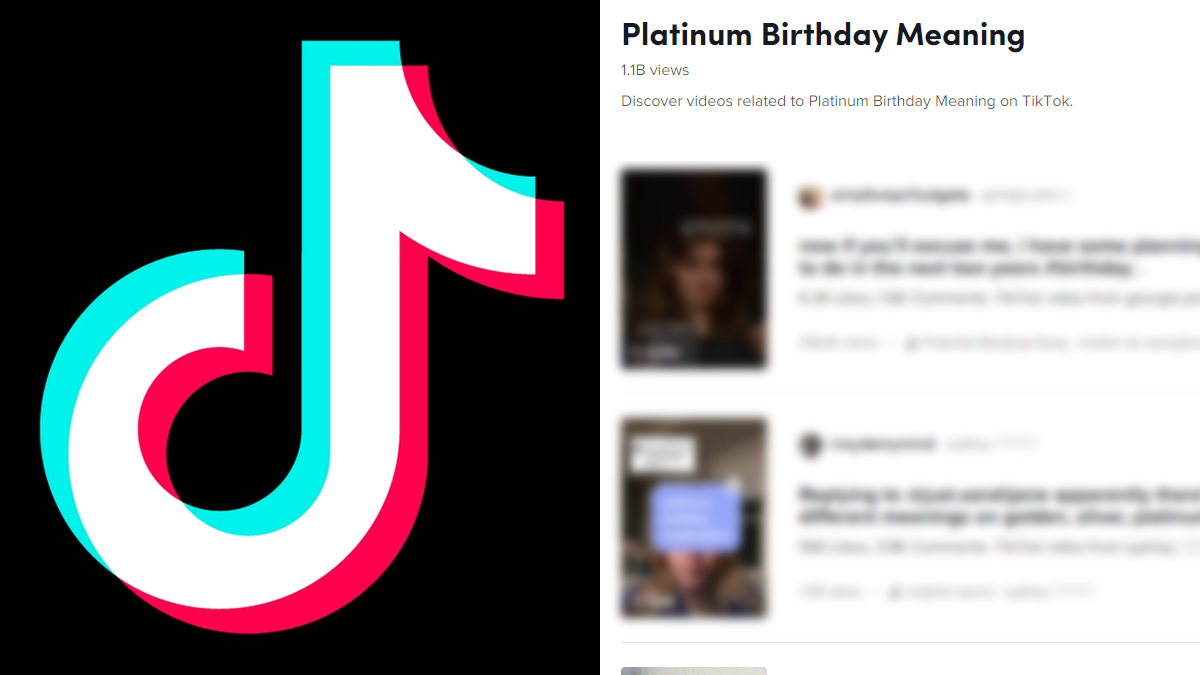This image is a screenshot taken from TikTok, formatted like a PC screenshot. The left half of the image prominently features the TikTok logo in a striking black square with aqua, pink, and white accents. To the right, against a white background, is a heading that reads, "Platinum Birthday Meaning," which has garnered a staggering 1.1 billion views. The caption invites users to "Discover Videos Related to Platinum Birthday Meaning on TikTok," confirming the platform source. Below this heading, there are two user comments, although both users' details are blurred and not readable. Each comment section includes a user photo above the comment text, with the comments themselves rendered in blue. The upper user image appears to be of a girl with dark hair, while the lower one shows a white rectangle, possibly indicating a piece of paper.